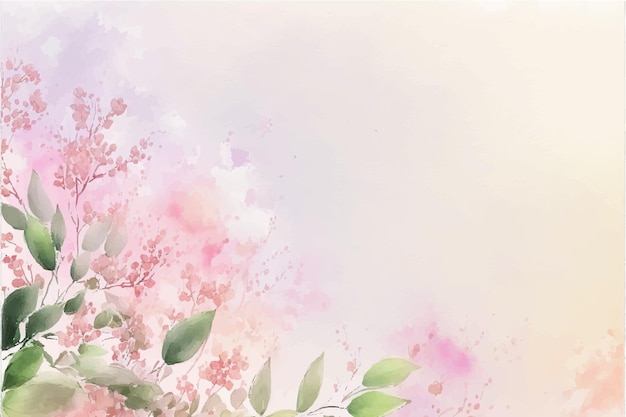The image, reminiscent of a desktop wallpaper or illustration, showcases a delicate watercolor scene. Starting from the bottom left and stretching to the top right, an array of meticulously modified and photoshopped leaves, in shades of dark and light green, frame the composition. Interspersed among the foliage are vibrant red buds and flowers with petals in varying hues of pink, subtly transitioning from pink to white. The backdrop is a soft, peachy color that seamlessly fades into lavender and pale purple gradients, creating an ethereal cloud-like effect. Light splotches of white and purple enhance the overall depth and texture, with additional soft pink splotches adorning the leaves at the bottom. The image has no text, allowing the intricate details and harmonious color transitions to stand out.